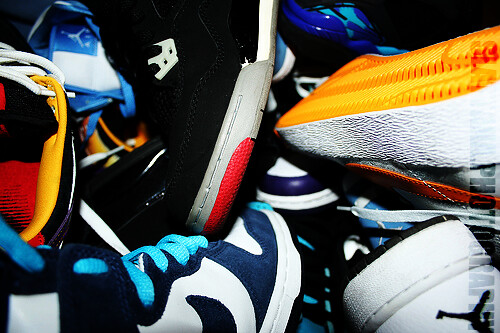This close-up photograph depicts a chaotic pile of approximately eight pairs of tennis shoes and sneakers, intermixed and overlaid so no single shoe is fully visible. The varied footwear showcases different parts: a heel here, an upside-down sole there, a top section covering the toes, a side view, and even an insole where the foot would rest. The assortment of colors is eye-catching, featuring red, orange, black, gray, white, turquoise, and several shades of blue. Although specific brands are hard to discern, there are suggestions of Nike designs among them. The shoes, adorned with shoelaces and adorned with multiple colored outlines, create a visually dynamic and layered composition, symbolized logos hint at familiar brands without clear identification, all contributing to the jumbled yet captivating scene of this footwear medley.